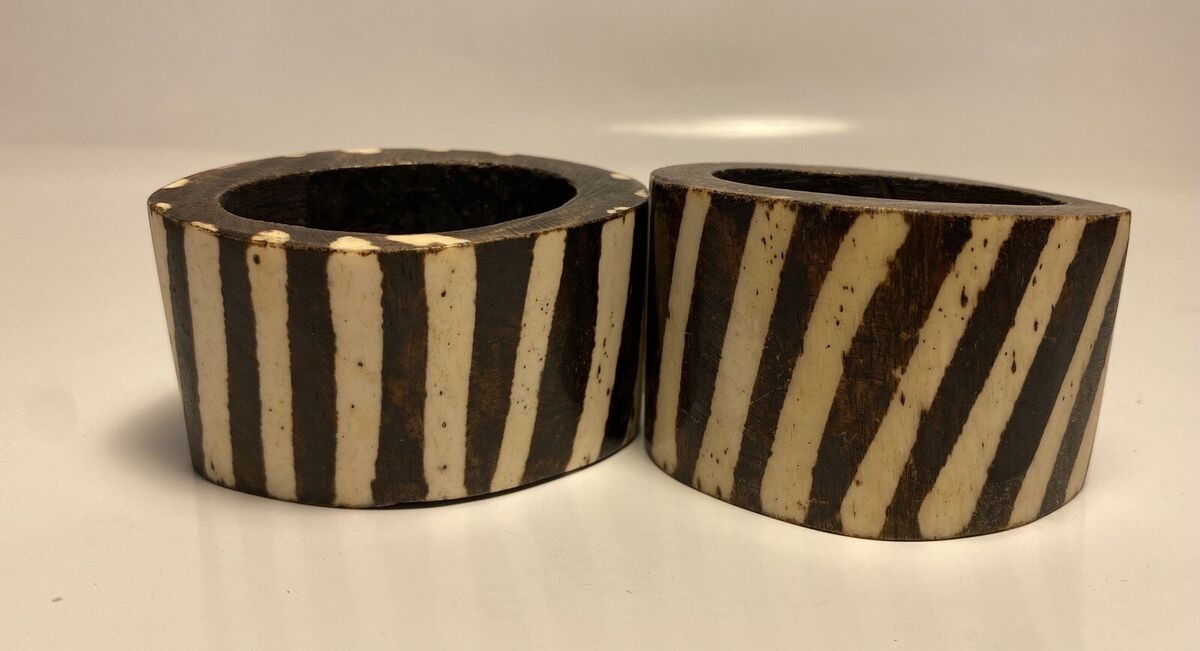The image depicts a close-up of two circular dessert items with a hollow interior, evocative of thick, oversized peanut butter cups. Both objects feature prominent brown and beige stripes that create a pattern resembling chocolate and vanilla swirls, enhancing their visual appeal. The item on the left appears slightly taller than the one on the right, and both are positioned centrally with ample space between them. The background of the image is a consistent, creamy beige hue, highlighting the desserts' intricate details and rich colors.